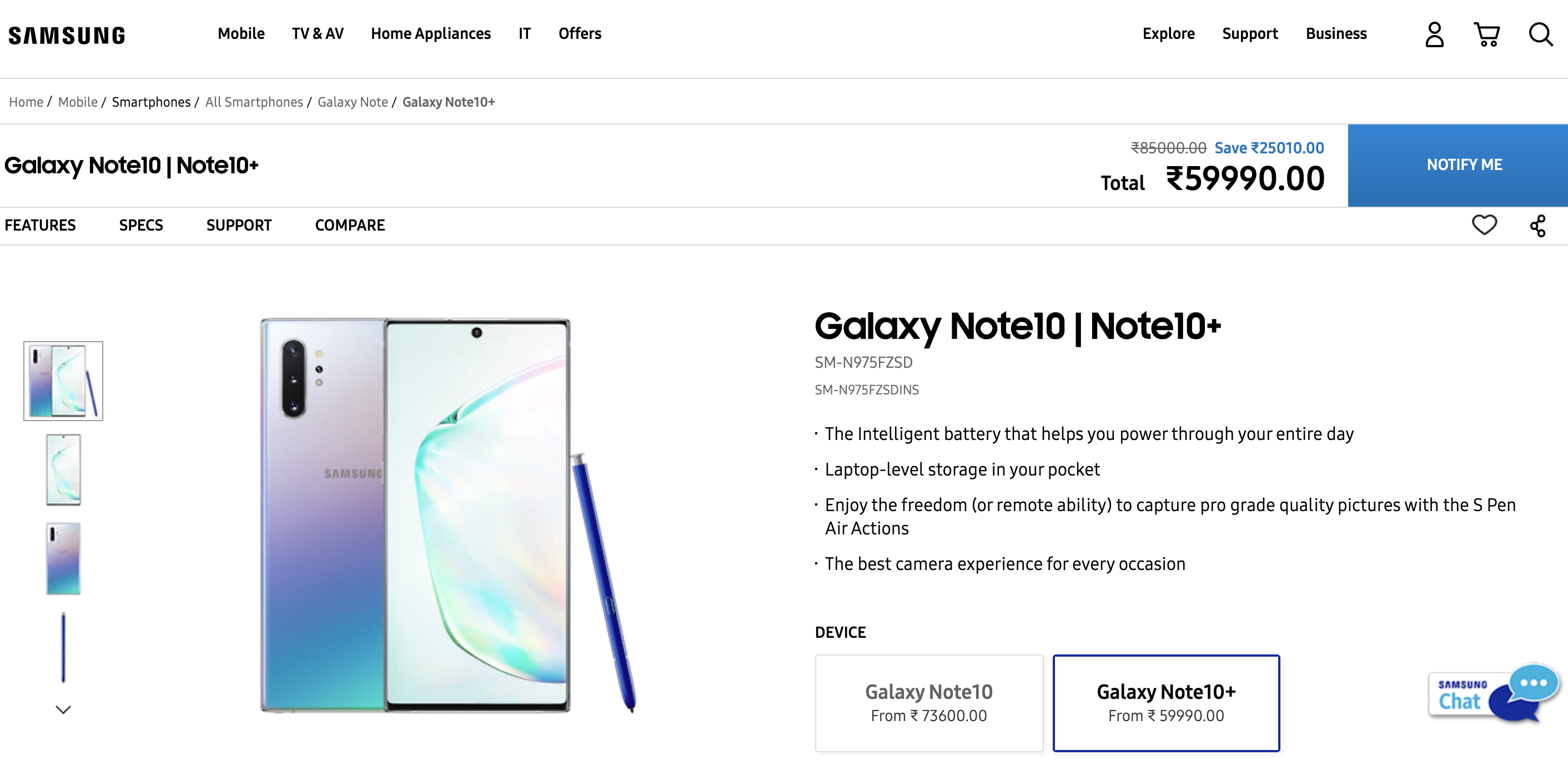A screenshot with a white background features the official Samsung website. The navigation bar includes top-level categories such as "Mobile," "TV & AV," "Home Appliances," "IT & Offers," "Explore," "Support," "Business," and icons for profile, shopping basket, and search.

Below this, the "Home Mobile Smartphones" section is highlighted in bold. There are subcategories listed, including "All Smartphones," "Galaxy Note," and under the "Galaxy Note" heading, the "Galaxy Note 10+" model is emphasized. The page provides various options like "Features," "Specs," "Support," and "Compare," accompanied by multiple slides showcasing the phone.

One specific slide features an image of the Galaxy Note 10+ with a blue stylus. The phone is prominently displayed with a price of $59,990.00, which is highlighted as a discounted price from the original $85,000.00 (scratched out). A savings amount of $250.10 is also indicated, although the currency symbol is unclear.

Below this, a blue rectangle button with "Notify Me" written in white awaits potential buyers. Additional highlights include mentions of the Galaxy Note series, specific model numbers "SM" followed by letters and numbers, and key features such as an intelligent battery designed for all-day use and ample storage comparable to a laptop. There are a couple more features listed that provide further details but are not fully visible in the screenshot.